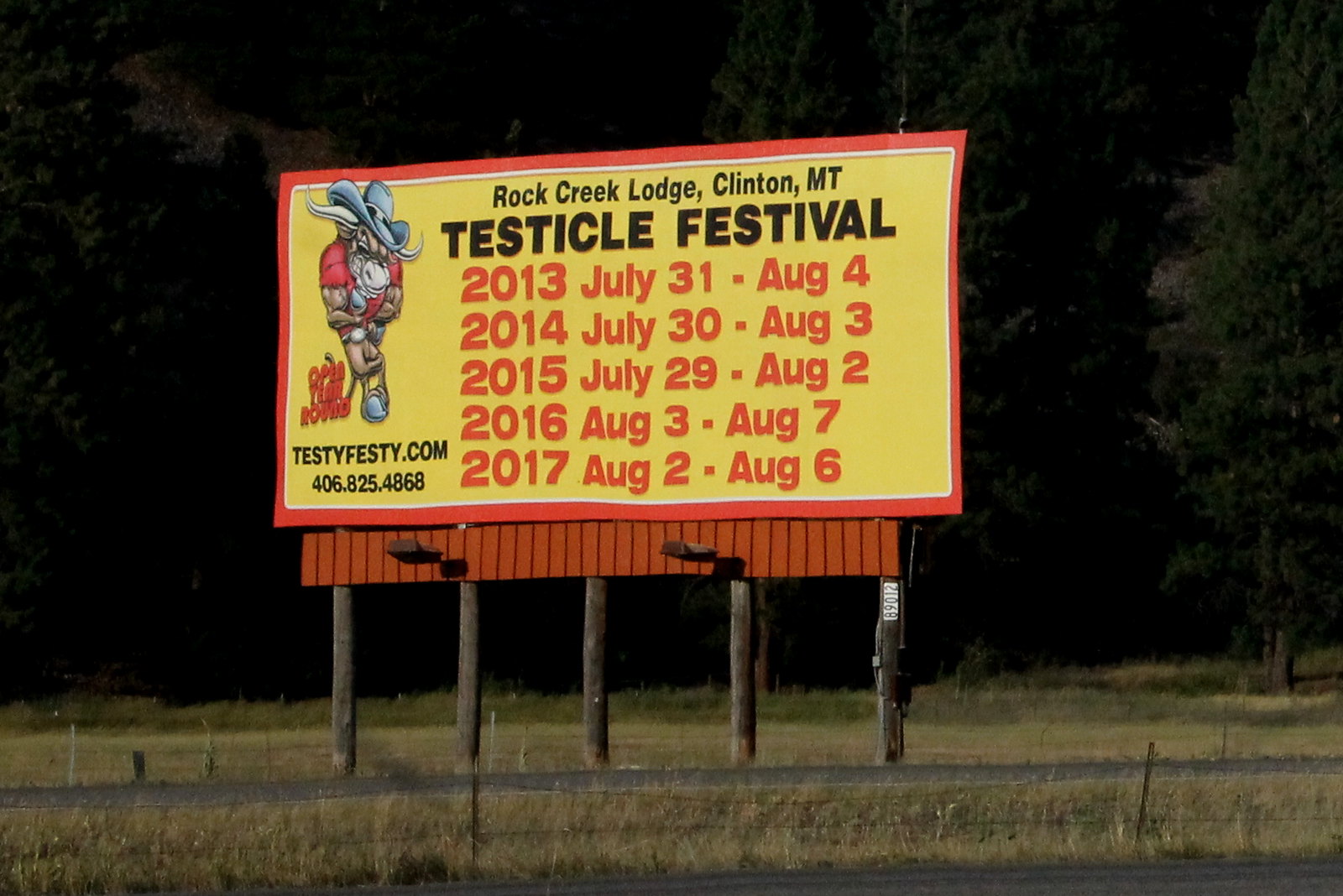In a real-life nighttime photograph, a large billboard situated about 10 to 12 feet off the ground is prominently displayed. The billboard, supported by five wooden posts, features a distinctive orange border and orange wooden strips along the bottom edge. The background color of the billboard is a bright yellow, which contrasts sharply with the dark night and encroaching greenery of a tree from the right. At the bottom of the image, there is a grassy area and a wooden fence, making up the lower 20% of the frame.

The upper left corner of the billboard showcases a cartoonish, muscular bull wearing a blue hat and a red T-shirt, with a fierce expression, likely serving as the festival's mascot. Next to the bull, in red letters, it reads "Open Year Round." Below the bull is the website “TESTIFESTI.COM” and the contact number "406.825.4868" in black capital letters.

Dominating the billboard, the main event being advertised is the "Rock Creek Lodge, Clinton, MT Testicle Festival," with "Testicle Festival" prominently written in large black capital letters. The event location and title are clearly stated in black at the top: "Rock Creek Lodge, Clinton, MT." The dates of the festival from 2013 to 2017 are listed in orange, with each year’s range placed directly below the other: 
- 2013: July 31st - August 4th
- 2014: July 30th - August 3rd
- 2015: July 29th - August 2nd
- 2016: August 3rd - August 7th
- 2017: August 2nd - August 6th

The bright yellow background and vibrant text make the billboard stand out against the almost entirely black nighttime setting, ensuring that the advertisement for the unique and humorously named "Testicle Festival" captures immediate attention.